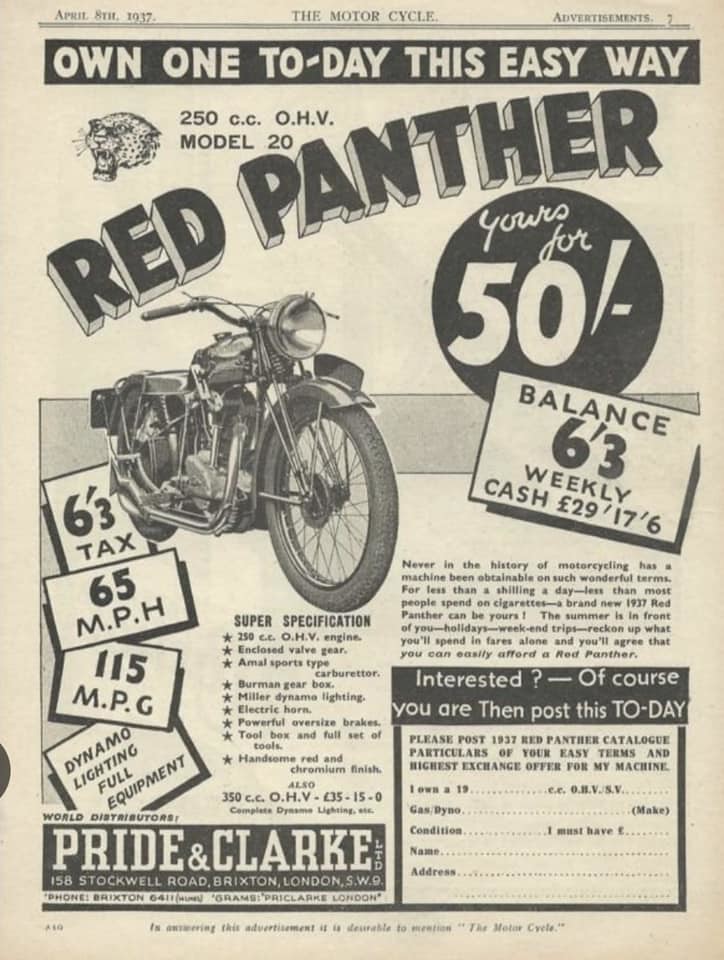This vintage advertisement from "The Motorcycle" magazine, dated April 8, 1937, promotes the Red Panther motorcycle. The ad boasts the new 250cc OHV Model 20, highlighting its affordability with the tagline, "Own One Today This Easy Way." The bike is priced at £50, with a balance payable at £6-3 weekly. Additional key features include a top speed of 65 miles per hour, an impressive 115 miles per gallon, and full dynamo lighting equipment. The ad visualizes the motorcycle alongside an illustration of a panther and breaks down costs, indicating a weekly payment structure and comprehensive details. At the bottom right corner, a bold box invites readers with "Interested? Of course you are. Then post this today." It offers purchasing instructions via World Distributor Pride and Clark, located at 156 Stockwell Road, London. A small form is included for potential buyers to fill out and send.